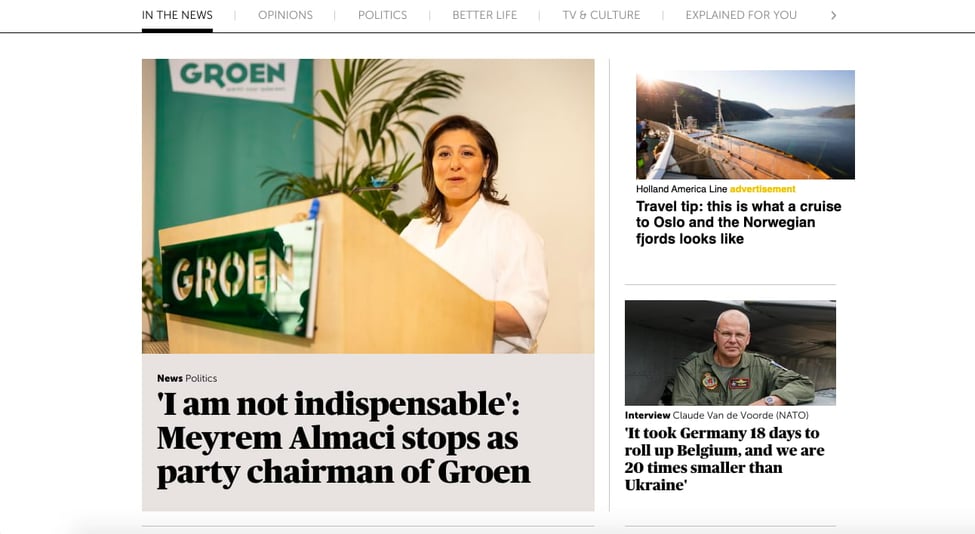This image depicts a web page from a news website, featuring six navigational tabs: "In the News," "Opinions," "Politics," "Better Life," "TV and Culture," and "Explained for You," followed by a right-facing arrow.

The main news article, prominently displayed to the left, features a woman standing at a wooden podium. The podium is made of light-colored tan wood. The woman, dressed in a white shirt, with brown hair, appears to be in a positive mood. Behind her, there is a palm plant and a green backdrop. The article's headline reads: "I am not indispensable: Meram Al-Machi steps down as party chairman of Growing."

To the right of this main article, there are two additional features. The first is an advertisement for Holland America Line, showing an image of the boat's deck, indicating travel tips about what a cruise to Oslo and the Norwegian fjords looks like. Below this ad is another article, titled "Interview with Claude Van de Voorde (NATO)," with a quote stating, "It took Germany 18 days to roll up Belgium, and we're 20 times smaller than Ukraine."